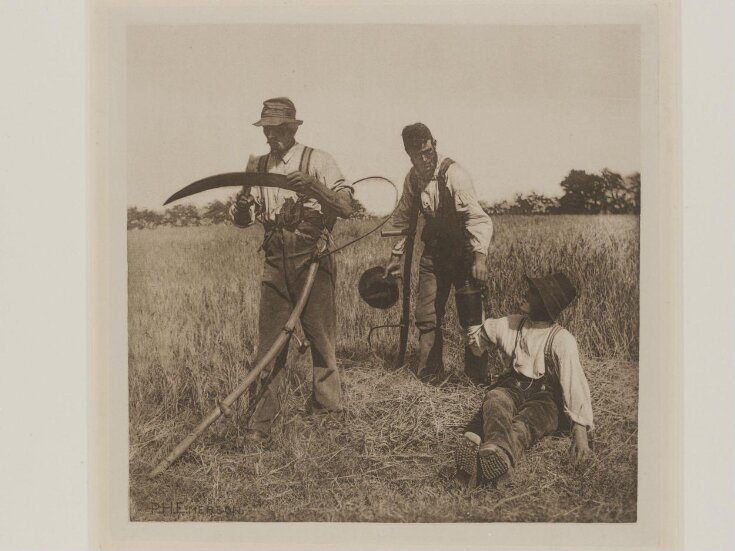An early 1920s photograph captures a group of three field workers taking a break in a vast wheat field under the bright midday sun. The central figure, a man with a mustache, is diligently sharpening a scythe, his concentration evident. To his right, a man with a shaded or possibly covered face, which could either suggest a shadow or indicate he is an African-American individual with a distinctive light chin, is also present. On the left, a third man holds his hat in hand, seemingly enjoying a moment of respite. They are surrounded by golden wheat stalks that stretch endlessly into the distance, broken only by a few trees far off on the right horizon. The sunlight casts sharp shadows directly under their feet, emphasizing the time of day and the intensity of their labor. This image captures not only the rustic simplicity of rural life but also serves as a poignant reminder of the hard work and diverse backgrounds of those who toiled in the fields.